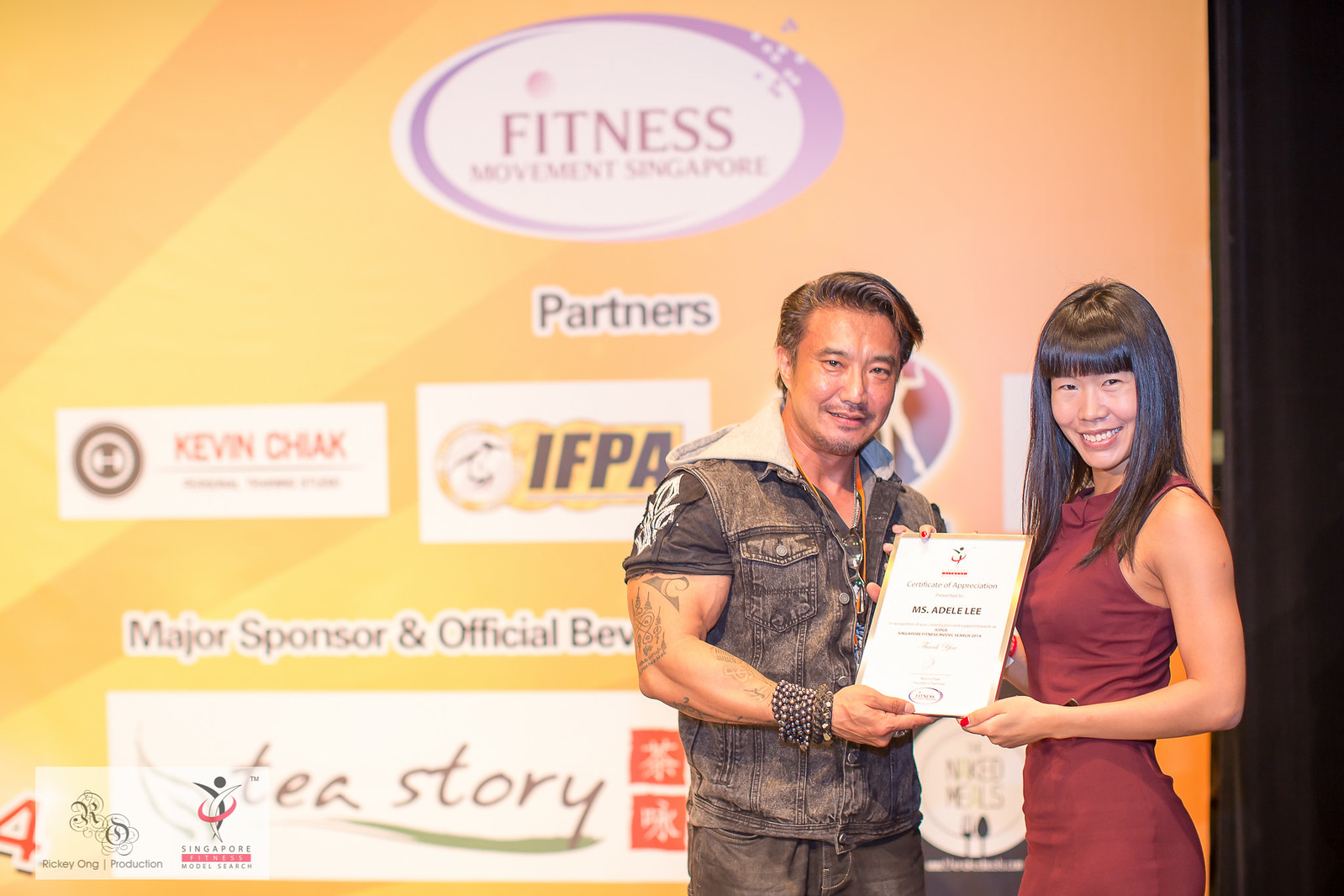Captured at the Fitness Movement Singapore event, this photograph features two individuals on a stage, framed by a yellow and orange banner with various sponsor logos, prominently including IFPA. The man, appearing to be in his 40s, has a distinct biker aesthetic with his slicked-back hair, a denim vest over a short-sleeved shirt, tattoos on his arms, and beaded bracelets. He sports a mustache and goatee and wears dark gray pants. Standing beside him is a woman in her 30s, identified as Ms. Adele Lee. She has long black hair with bangs and is dressed in a burgundy dress. Both are smiling as they hold a Certificate of Appreciation, with Adele Lee seemingly presenting it to the man. The banner behind them highlights the event's affiliation with Fitness Movement Singapore.